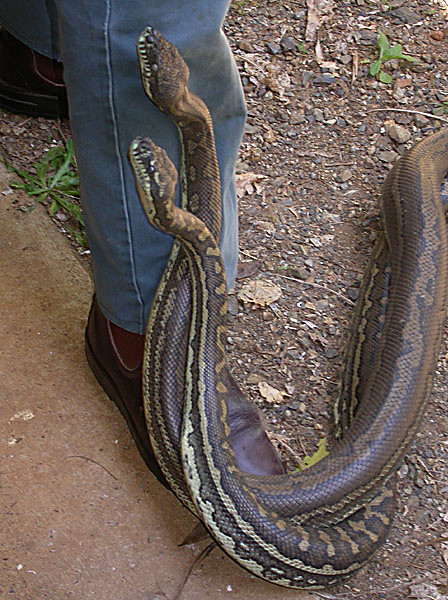In this detailed photograph, two large pythons, displaying a mix of brown and beige patterns, are intertwined and climbing up a man's leg. The man, dressed in blue jeans and dark tan leather shoes, stands with his right foot partially on soil and partially on a brick pavement. The scene is outdoors, in daylight, possibly overcast, with a background showing a ground scattered with stones, rocks, twigs, and small patches of grass and plants. The pythons, starting from the man’s boots, have entwined themselves and are progressively crawling upwards, having reached just below his knee. The man appears calm as the sizeable snakes, which are not venomous but still imposing, advance up his leg. His body is visible only from the waist down.